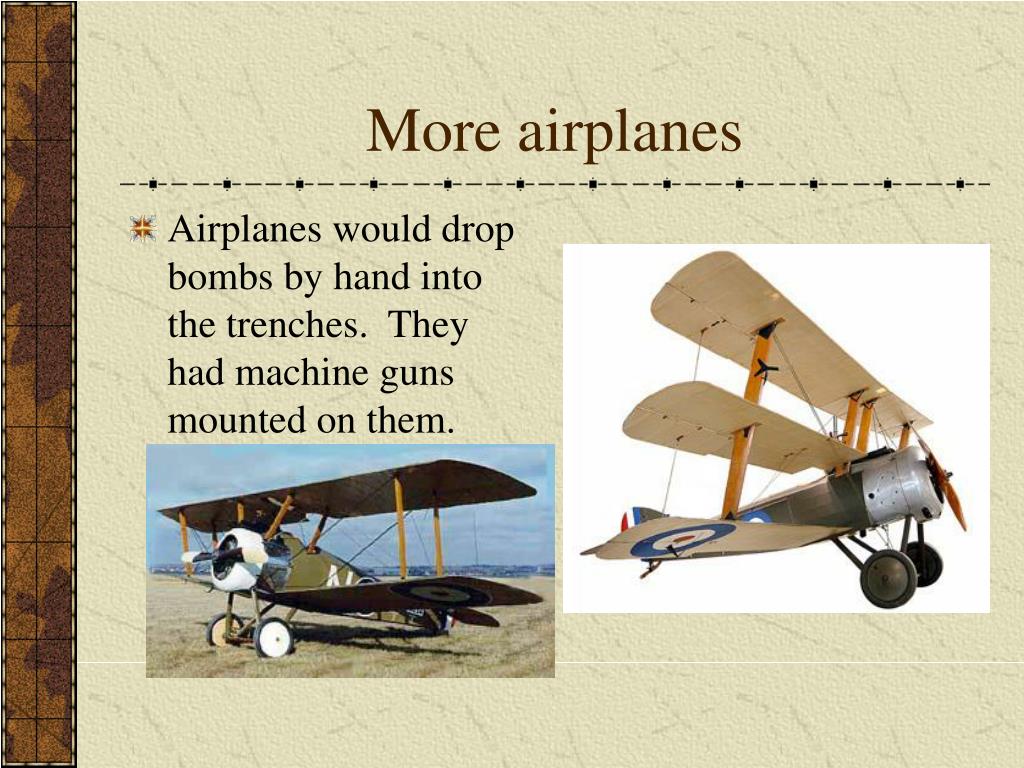The image resembles a Microsoft PowerPoint slide with a background featuring a beige color and a narrow brown strip on the left side, possibly resembling a binding with a leaf pattern. The slide is titled "More Airplanes" at the top in brown lettering. Below the title, on the left side, a small paragraph in black font against the greenish, parchment-like background reads: "Airplanes would drop bombs by hand into the trenches. They had machine guns mounted on them."

Beneath this text, there is a color photograph of a moss-green biplane, identifiable by its single engine and the propeller mounted at the nose. This early 20th-century aircraft features two wings, one above and one below the fuselage, connected by struts, with a prominent cockpit in the center.

To the right of the text and the first image, a second image depicts a triplane, predominantly dark gray with a silver nose. The triplane, which appears to be a model, showcases three sets of wings with struts, one below and two above the fuselage. A notable detail is the symbol of the Royal Air Force—a blue circle with a white circle inside and a red dot in the center—visible on the underside of the lowest wing.

Both aircraft shown, one a biplane and the other a triplane, are from the World War I era, exemplifying the types of planes used to drop bombs by hand into enemy trenches and equipped with machine guns. The distinct colors and designs, including the blue, white, and red target insignia, highlight their historical significance and specific roles in early aerial warfare.